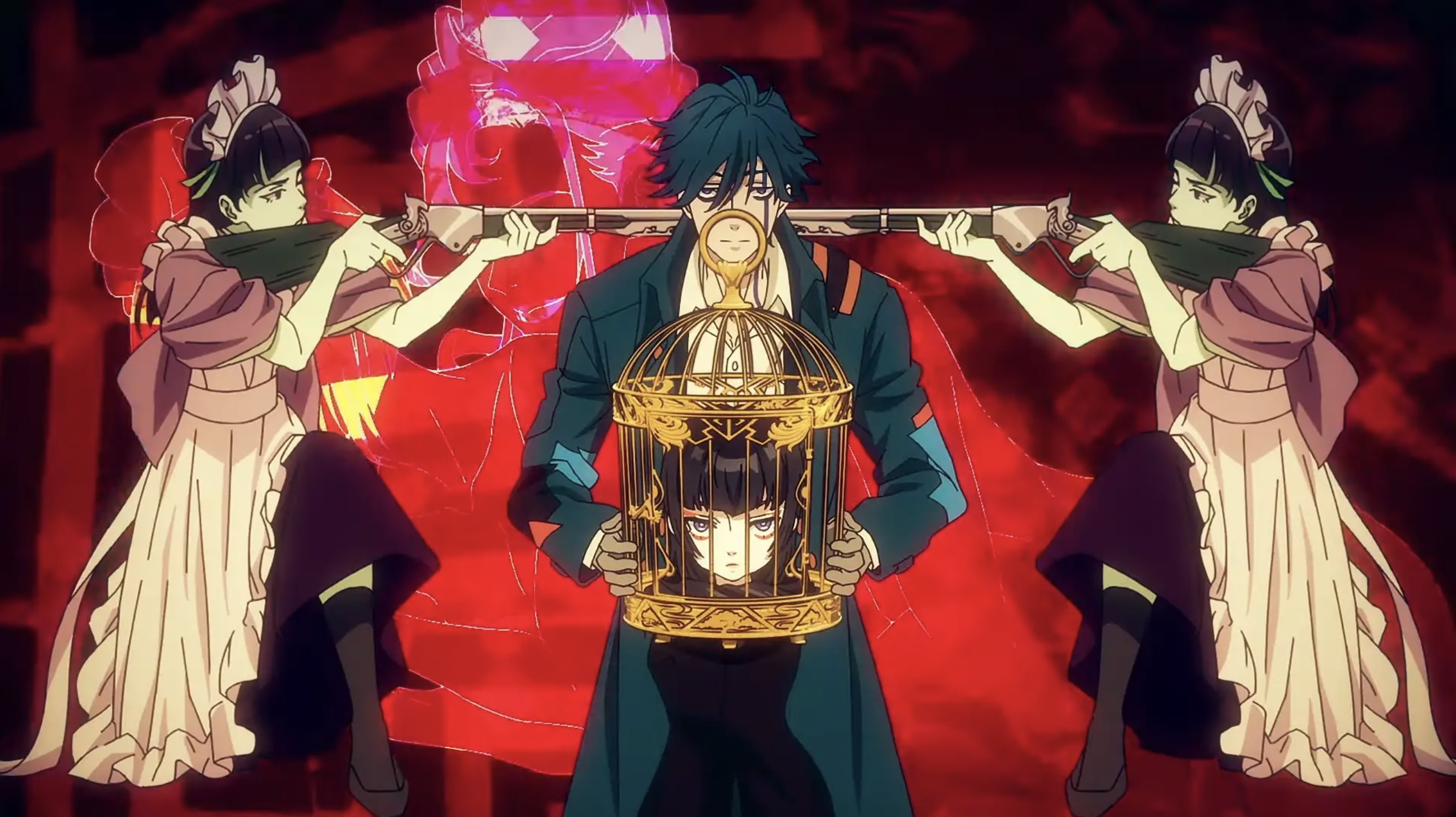The image depicts a tense anime scene featuring three characters in a striking, futuristic yet early 1900s-inspired setting. Two women, dressed in traditional maid outfits with frilly aprons and headbands, kneel on opposite sides of the image, each aiming a silver and black rifle directly at the other, their weapons intersecting mid-frame behind the head of a central male figure. This man, with short, dark hair partially covering his eyes, stands in the foreground, wearing a long trench coat adorned with orange, blue, and red patches, over a white button-up shirt. His expression is neutral as he holds a large, gold birdcage across his chest, containing the stern, short-haired head of a woman, who appears to be questioning the situation. The backdrop is a vivid red and black schematic with neon pink accents, adding to the dramatic and surreal atmosphere of the scene.